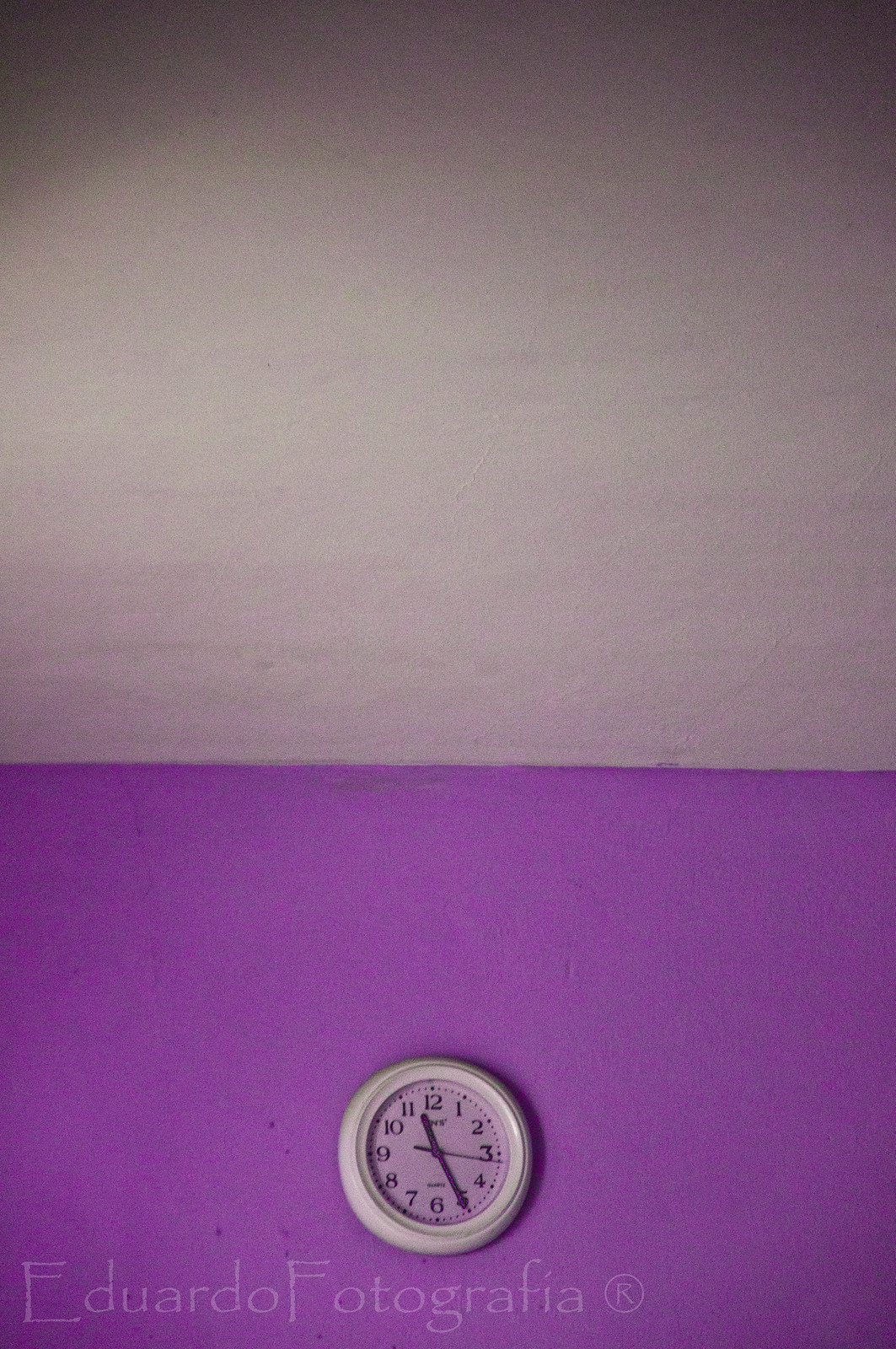The image depicts a simple, minimalist interior view captured by Edward Fotografia. We are looking up at the intersection of a medium purple wall and an off-white to light grayish ceiling, where the transition occurs roughly 45% up from the bottom of the image. Central to the composition is an analog clock with an off-white plastic circular frame, positioned towards the bottom center of the wall. The clock’s hands indicate the time is approximately 5:17. Overall, the ceiling is plain with no distinctive features, while the wall below is uniformly purple, creating a straightforward yet striking visual.